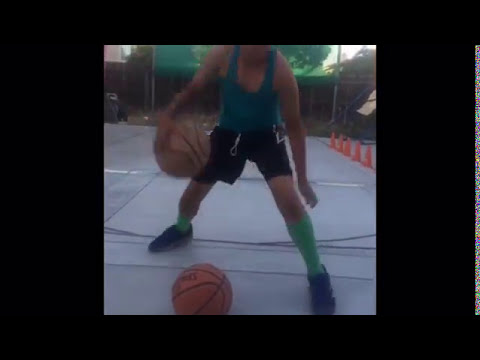The image portrays a person, depicted from the neck down, engaged in a basketball drill on an outdoor court. The individual appears to be an African American male wearing a turquoise tank top, black shorts, vibrant lime green knee-high socks, and black shoes. He is actively dribbling a standard brown basketball with black seams in his right hand. Positioned near his right foot is another basketball lying on the ground, hinting at a possible double-dribbling exercise. The court itself is gray and occupies the bottom and middle two-thirds of the frame, while a series of five orange cones line the right side of the image, suggesting a drill setup. In the background, a tall, dark brown fence encloses the court. The visual focuses on basketball practice, emphasizing the highly dynamic action of dribbling amidst a structured training environment.